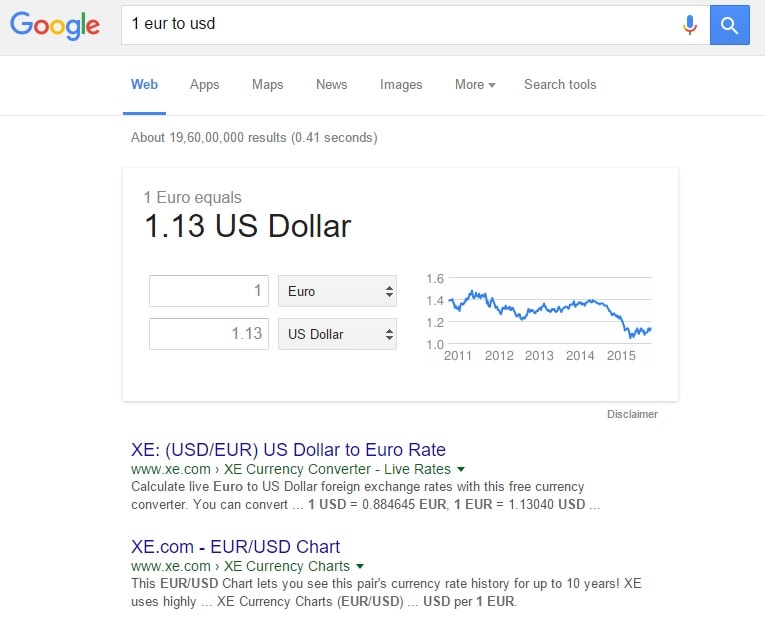The image depicts a Google search results page for currency conversion. At the top, familiar Google branding and its search bar are visible. Someone has searched for "1 EUR to USD," indicating they want to convert 1 Euro to US Dollars. The search icon is present in the search bar. Below, multiple headings such as Web, Apps, Maps, News, Images, and a drop-down menu labeled "More" are shown alongside "Search Tools." The "Web" tab is highlighted.

In gray text, the page notes approximately 19,600,000 results. A conversion box prominently displays the answer: "1 EUR equals 1.13 USD" in bold black letters. This section features interactive components: a small input box containing the number "1" next to the label "EUR" with arrows for selecting different currencies. Below, another input box allows users to enter different amounts to convert. Adjacent to this is a drop-down menu for selecting the target currency. To the right of these boxes, a chart illustrates the conversion rate trends over time.